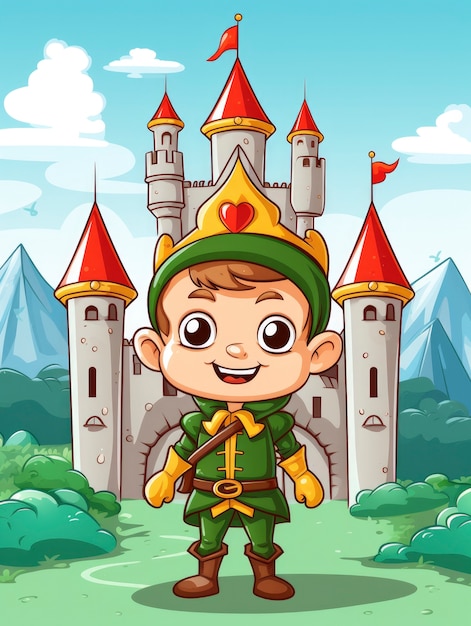An animated cartoon image showcases a young elf-like character with wide, round black eyes and a big smile. Dressed in green clothing, yellow gloves, and brown shoes, the character also sports a green hat adorned with a gold crown featuring a small heart. He stands on lush green grass with bushes around, and the background reveals a grand castle made of stone with red turrets and yellow bases. The castle's design is enhanced by a couple of red flags atop the turrets. Behind the castle, a serene expanse of blue sky dotted with puffy white clouds frames the scene, coupled with the majestic, snow-covered peaks of distant mountains.